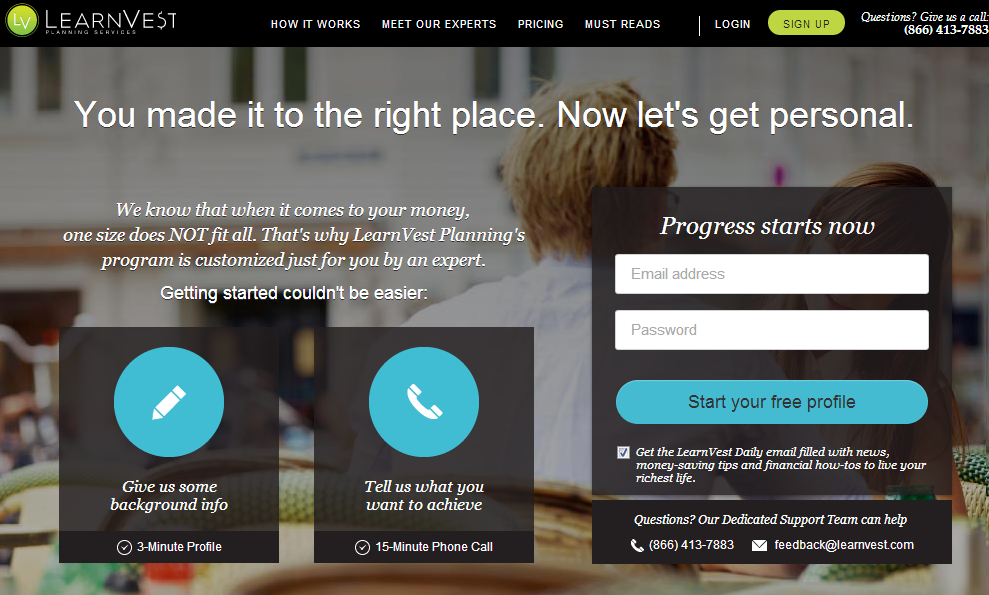**Detailed Caption:**

This screenshot showcases the homepage of the LearnVest website. At the top, the LearnVest logo, in a lime green hue, is prominently displayed alongside navigation tabs such as "How It Works," "Meet Our Experts," "Pricing," and "Must Reads." Options to "Log In" or "Sign Up" are also available in this top banner.

In the background, an image features a couple seated outdoors in a vibrant urban setting, sharing a meal and enjoying the picturesque cityscape. This adds a personal and inviting touch to the website's design.

The interface mainly consists of text elements, interspersed with logos and icons. Grayscale tones dominate the color palette, accented with a teal blue used for various interactive buttons. Black banners provide a sharp contrast, adding to the sleek visual appeal.

Centered on the page, a welcoming message reads: "You made it to the right place. Now, let's get personal. We know that when it comes to your money, one size does not fit all." This emphasizes the customized financial planning services offered by LearnVest, designed to be tailored by experts to meet individual needs.

For further assistance, there's a prominently displayed customer service number: 866-413-7883, ensuring users can easily access help and support if needed. Overall, the design and content aim to provide a user-friendly and personalized experience for managing finances.